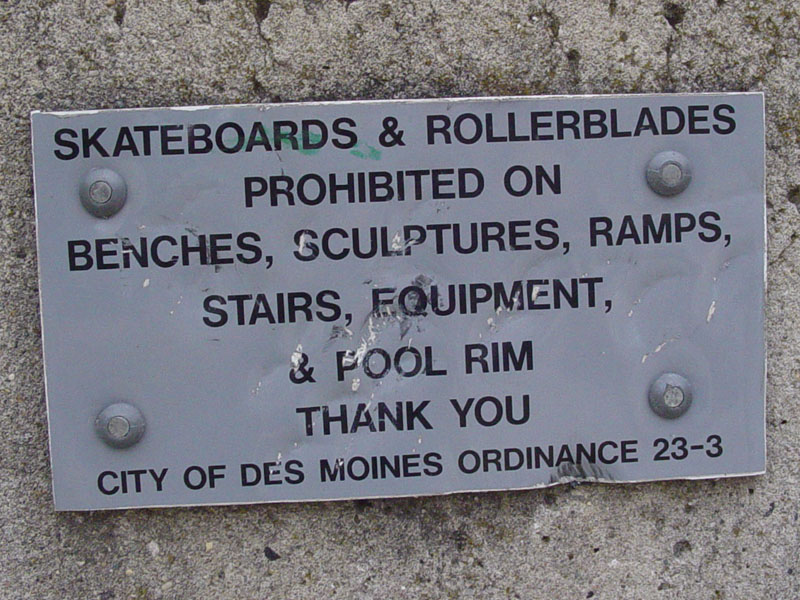The image depicts a weathered metal plaque mounted diagonally on a worn stone or concrete wall. The plaque, affixed with four bolts—two on the top corners and two on the bottom corners—features uppercase black text that reads: "SKATEBOARDS AND ROLLERBLADES PROHIBITED ON BENCHES, SCULPTURES, RAMPS, STAIRS, EQUIPMENT, AND POOL ROOM. THANK YOU. CITY OF DES MOINES, ORDINANCE 23-3." The sign appears old and has sustained various forms of damage; it is dented at the bottom right corner, scratched and scuffed around the middle and right side, and marred with some unintended green paint near the word "skateboards." This suggests frequent use of the area by skateboarders and rollerbladers despite the prohibition.